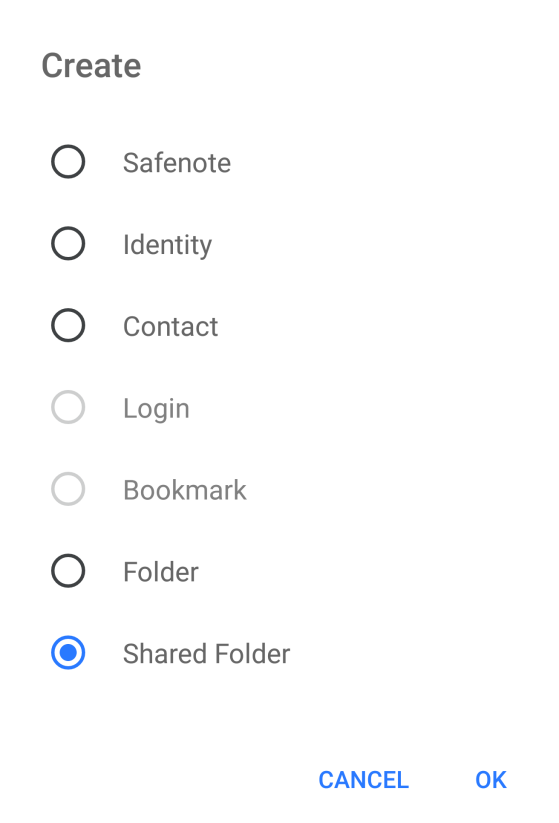In this image, the interface appears to be from a software application, likely related to settings or organization tools, all set against a clean, white backdrop. At the upper-left corner, the word "Create" is prominently displayed in black text. Below "Create," there are several labeled icons arranged vertically:

- The first icon is a white circle outlined in black with the label "Safe Note" to its right.
- Below that, a similar white circle outlined in black is labeled "Identity."
- The next icon is a white circle outlined in black with the label "Contact."
- Following this, there is a white circle outlined in a light shade of gray, labeled "Login."
- Another white circle outlined in a light gray shade is labeled "Bookmark."
- A subsequent white circle outlined in black is labeled "Folder."
- The final icon in the series is a white circle with a blue circle in the middle and outlined in blue, labeled "Shared Folder."

At the bottom left of the interface, the word "Cancel" is displayed in blue text, followed by a space. Next to it, also in blue text, are the letters "O" and "K," signifying an "OK" button. This detailed layout suggests a user-friendly design aimed at providing easy access to various organizational functionalities.